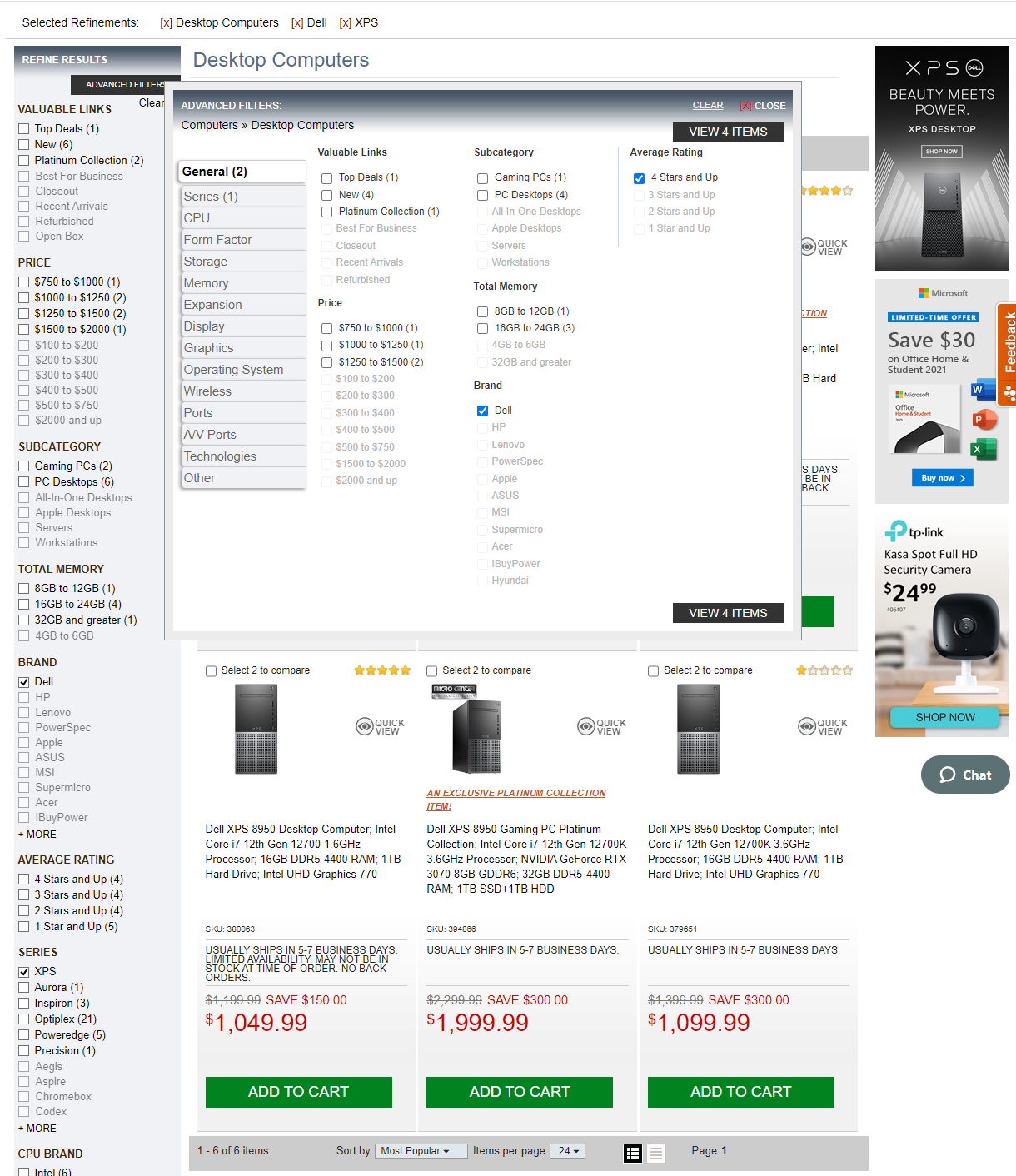A cluttered webpage dedicated to the sale of computer parts is displayed. The website prominently features various Dell computer models, alongside options from other brands like HP, Lenovo, PowerSpec, Apple, Asus, MSI, Supermicro, Acer, and iBUYPOWER. Categories such as "Gaming PCs" and "PC Desktops" are organized on the left-hand side, which also includes filters for "Top Deals," "New Arrivals," and a "Platinum Collection." Prices of the listed products range between $750 and $2,000.

Highlighted deals comprise the Dell XPS series, featuring models like the Dell XPS 8950 desktop computer with Intel Core i7, 12th Gen 12700 processor, and Intel UHD Graphics – evaluated as having an insufficiently high-performance processor. Another example is the Dell XPS Gaming Platinum model, equipped with Nvidia RTX 3070 graphics. 

Memory options span from 8GB to 32GB, and users can sort products by average ratings, which range from 4 to 5 stars. Models include Dell's XPS, Aurora, Inspiron, OptiPlex, and Vostro series. The webpage suggests further Dell models at the bottom, priced between $1,049.99 and $1,999.99, all criticized for their perceived poor value. 

Users have the ability to add these computers to their cart directly from the listing. Despite the array of available brands and specifications, the selection is described overall as offering underwhelming deals.